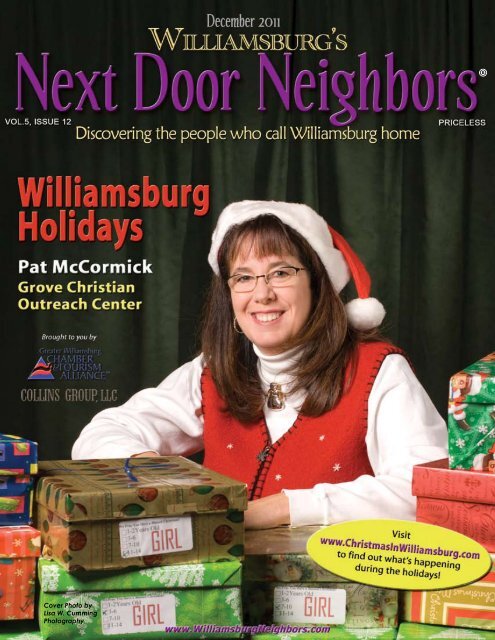The December 2011 cover of Williamsburg's Next Door Neighbors magazine, Volume 5, Issue 12, features the tagline "Discovering the People Who Call Williamsburg Home" at the top. The magazine title "Next Door Neighbors" is displayed in purple text, while "Williamsburg's Holidays" appears in red print. In focus is a friendly-looking woman with long brown hair and glasses, smiling warmly at the camera. She is adorned in a festive Santa hat, a white turtleneck, and a red vest decorated with small stars. In front of her are an array of Christmas presents marked for girls. The cover also highlights an article on Pat McCormick from the Grove Christian Outreach Center. Additionally, there's a yellow blurb directing readers to visit www.christmasinwilliamsburg.com for information on holiday events.